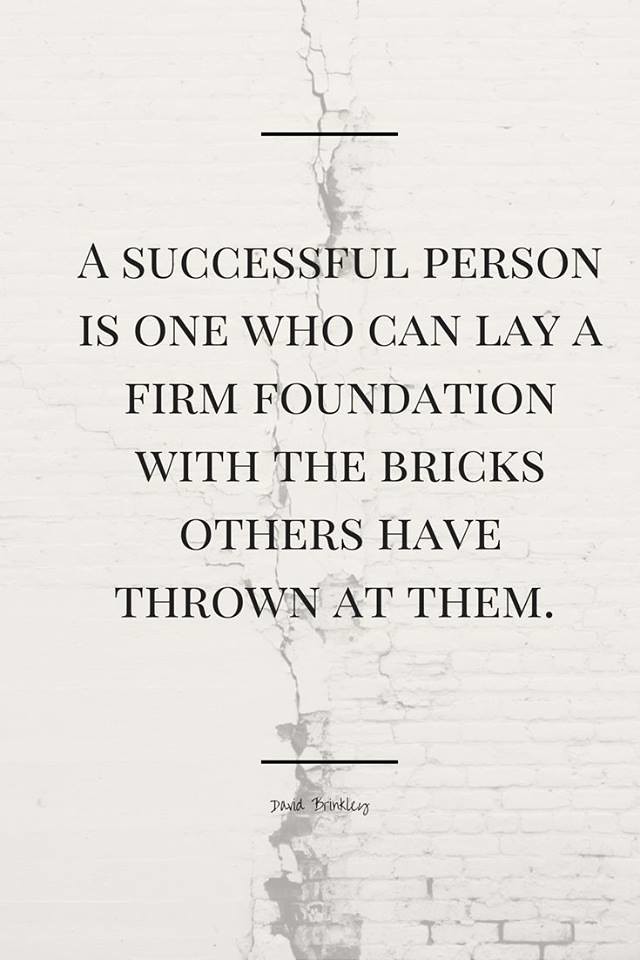The image appears to be a motivational poster with a predominantly white background designed to resemble a decaying or cracked brick wall. Subtle lines and cracks within the white space enhance this rugged, structural appearance. 

Centered in the image, inscribed in bold, black capital letters, is the inspirational quote: "A SUCCESSFUL PERSON IS ONE WHO CAN LAY A FIRM FOUNDATION WITH THE BRICKS OTHERS HAVE THROWN AT THEM." This text is divided into multiple lines to maintain balanced alignment within the composition.

A thin, black horizontal line runs across the top and the bottom of the quoted text, further segmenting the layout. Beneath the bottom line, the name of the quote’s author, "David Brinkley," is elegantly signed in black, providing attribution to the well-known journalist.

The overall design evokes a sense of resilience and strength, visually symbolized by the distressed brick wall, underscoring the message of overcoming adversity with fortitude.